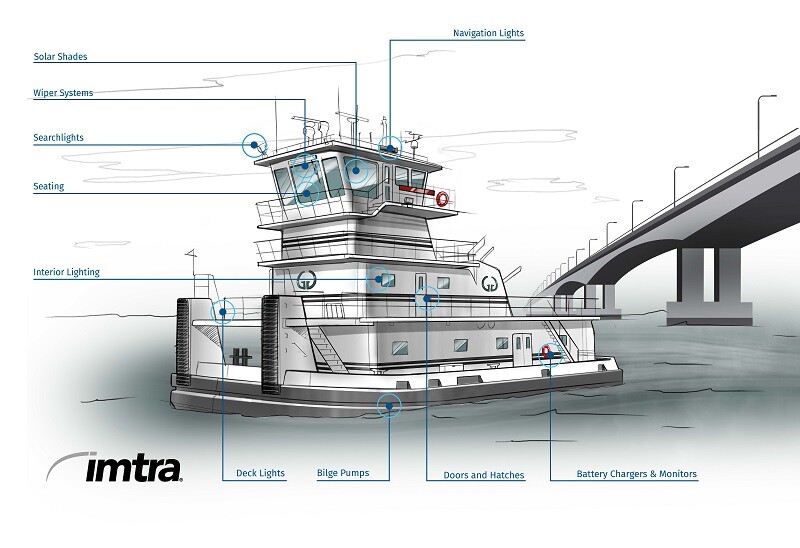The image is a detailed, cartoon-style graphic of a boat, possibly a ferry, depicted in a predominantly gray, white, black, and blue color palette. The boat is floating on grayish water near a concrete bridge on the right side of the image. It features multiple decks leading up to a glass-enclosed tower area at the top. Numerous white lines extend from various parts of the boat to clear, labeled descriptions of its components, including solar shades, wiper systems, searchlights, seating, interior lighting, navigation lights, deck lights, bilge pumps, doors and hatches, and battery chargers and monitors. The bottom left corner of the image is marked with the label "IMTRA," indicating a possible manufacturer or related brand.